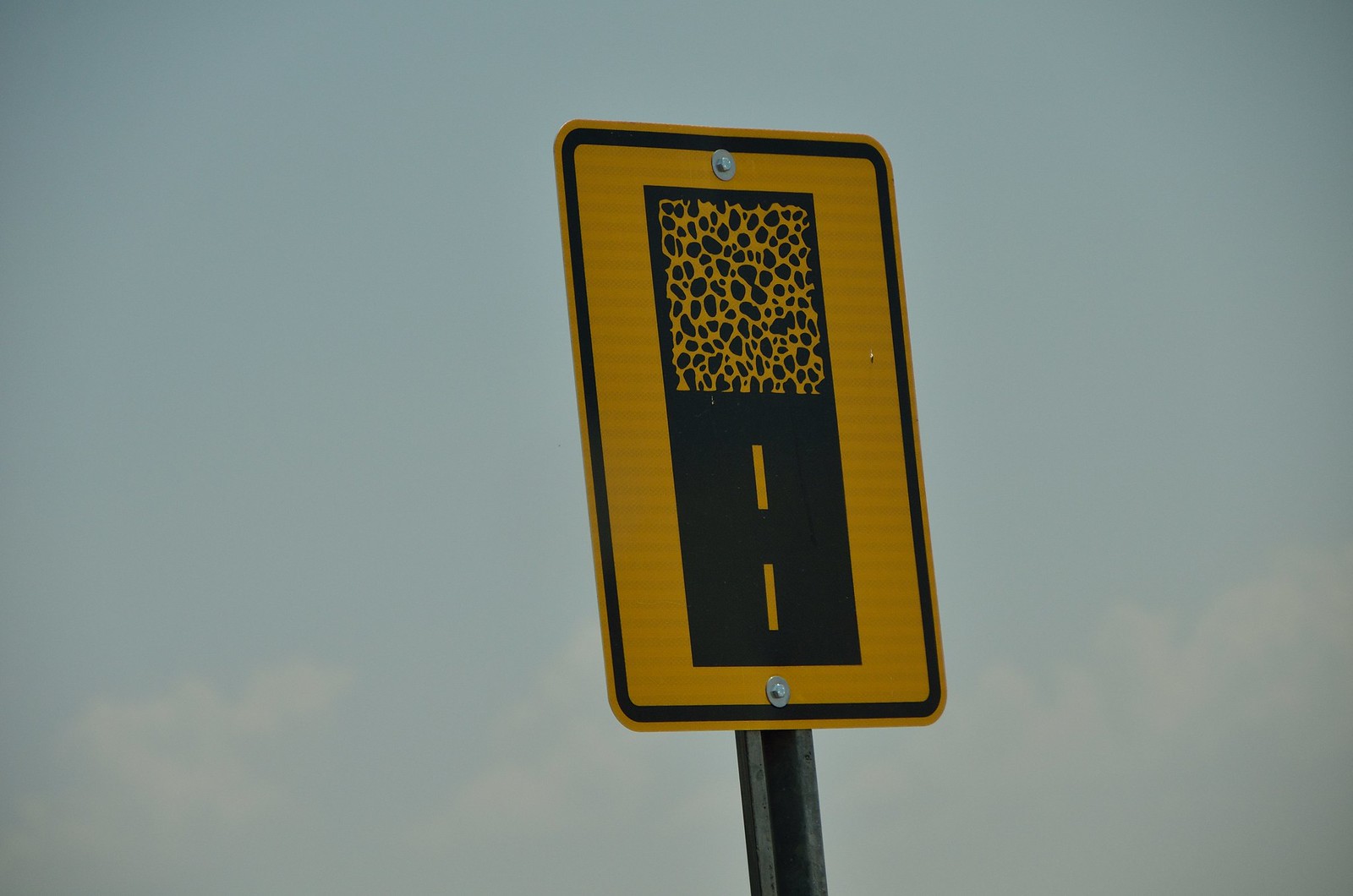This image depicts a clear, high-quality close-up of a street sign set against a background of a predominantly blue sky with a few light clouds. The sign is rectangular and primarily yellow, with a black border and another yellow band inside the border. A black rectangle occupies the lower section of the sign, featuring two parallel dashed lines running from the bottom to the top, indicative of a divided roadway. Above this, within the black rectangle, is a yellow square filled with black dots, possibly representing an upcoming transition to a gravel or cobblestone road. The sign is mounted on a pole, which is slightly visible at the bottom of the frame. The overall scene is bathed in daylight, enhancing the visibility of the sign's details.